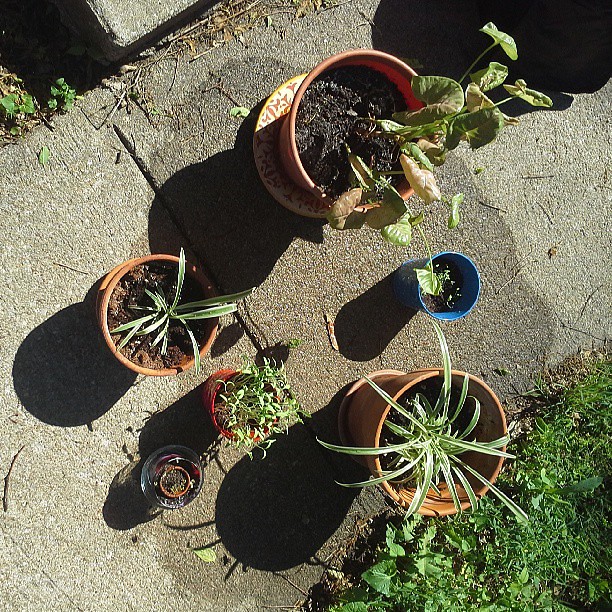This is an overhead, color photograph of a sunny sidewalk in front of what is likely someone’s home. The typical concrete sidewalk, segmented by clean-cut lines, is adorned with several potted plants arranged on drainage saucers. There are five main pots: three large, reddish-orange clay pots, a smaller blue pot, a tiny red pot, and an even tinier glass container. The largest orange pot houses a substantial plant, while two other orange pots contain long, skinny spider plant-like leaves. The blue pot's contents are unclear, but the red pot has short sprouts emerging from it. The glass container appears to be attempting to grow something as well. Scattered leaves and sticks can be seen on the sidewalk, with a patch of green grass in the upper left and bottom right corners of the photograph. The concrete sections around the pots show wet patches, suggesting that the plants have been recently watered. None of the plants display flowers, and the entire scene is devoid of people, animals, or buildings.